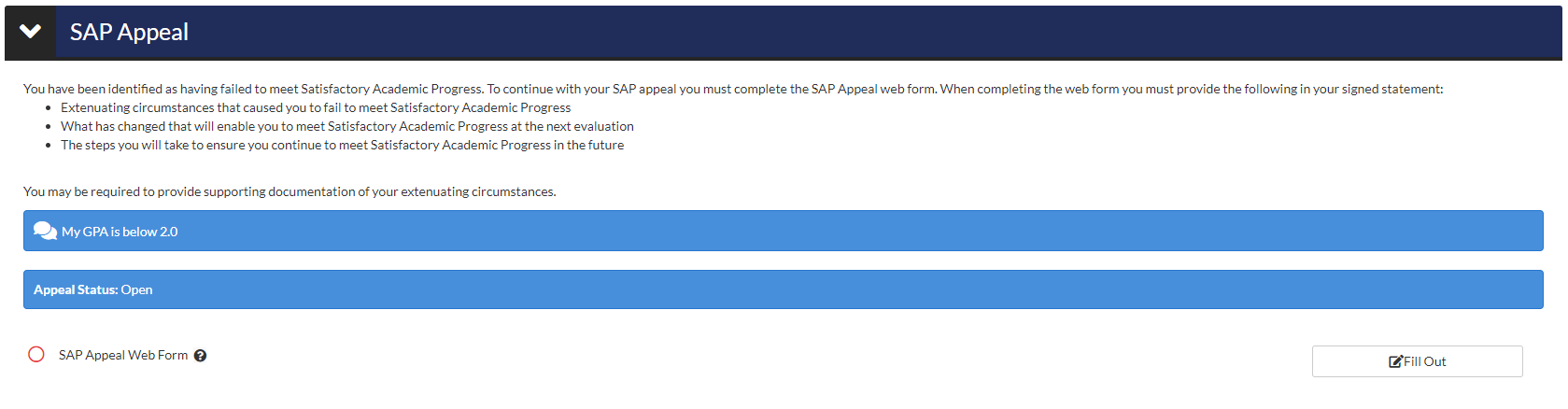Here's a detailed, cleaned-up descriptive caption for the provided image:

---

**Screenshot Description:**

The image depicts a screenshot of a website, primarily focused on a notification regarding an SAP (Satisfactory Academic Progress) appeal.

**Header Section:**
- At the top of the webpage, there is a dark blue rectangular bezel. On the left side of this bezel is a black square, positioned on its edge, containing a bold, white downward-pointing arrow.
- Within the dark blue rectangle, the acronym "SAP" is prominently displayed in all caps, followed by the word "Appeal" with only the first letter capitalized.

**Main Notification:**
- Underneath this header is a white rectangle containing the following message in black text:
  - "You have been identified as having failed to meet satisfactory academic progress. To continue with your SAP appeal, you must complete an SAP appeal web form. When completing the web form, you must provide the following in your signed statement:"
  - This section then continues with bullet points detailing the required information:
    - "Extenuating circumstances that caused you to fail to meet satisfactory academic progress."
    - "What has changed that will enable you to meet satisfactory academic progress at the next evaluation?"
    - "The steps you will take to ensure you continue to meet satisfactory academic progress in the future."
  - The message concludes with a note: "You may be required to provide supporting documentation of your extenuating circumstances."

**Mid-Section:**
- A mid-blue rectangle is displayed below the main notification. This compartment includes two sections:
  - To the left, white chat bubble icons are shown.
  - To the right, in bold white text, it states: "My GPA is below 2.0."

**Additional Information:**
- Below the mid-blue rectangle is another similar rectangle with more prominent, bold white text. It reads: "Bill Status: Open."

**Footer Section:**
- In the white space outside the blue rectangles, there is a red circle positioned towards the right. Next to the red circle, in regular black text (not bold), the following information is provided:
  - "SAP Appeal Web Form."
- Additionally, a black circle containing a white question mark is placed nearby, suggesting the availability of further information or help related to the form.

---

This thorough caption provides clear and comprehensive details about the contents and layout of the screenshot.